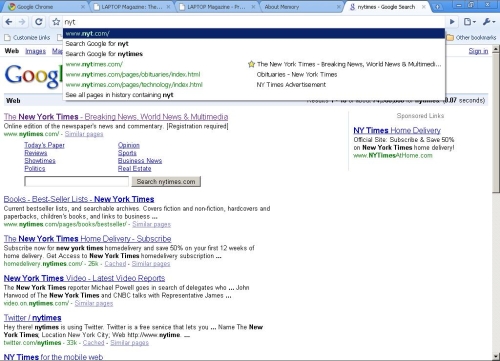The image is a screenshot of a Google search performed in Google Chrome. The Google logo, prominently displayed at the top, features its iconic colors of blue, red, yellow, and green. Below the logo is the search bar, where someone has typed "NYT." The search bar is white with a blue underline.

The search results pertain to the New York Times (NYT), listing several sections such as Breaking News, World News, and Multimedia. Additional links include categories like Bestsellers, Home Delivery, Subscribe, New York Times Video, and Twitter. There is specific mention of "New York Times for the mobile web."

On the right side of the search results, there is a panel with information regarding New York Times Home Delivery. A drop-down box appears, indicating suggestions for "NYT.com" with a yellow star next to "The New York Times, Breaking News, World News, and Multimedia." This drop-down also includes categories like obituaries and advertisements related to the New York Times.